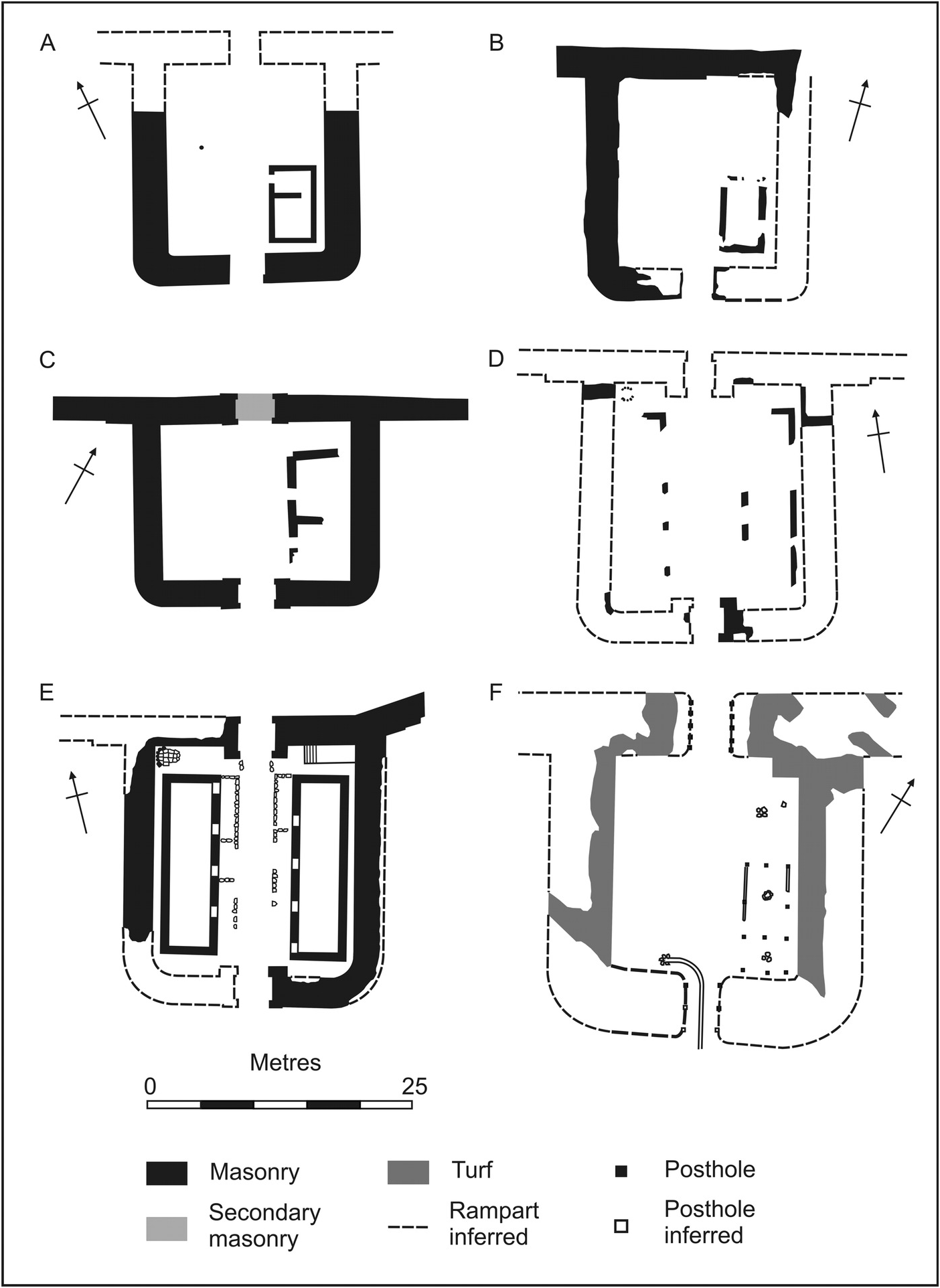This architectural blueprint is divided into six sections labeled A, B, C, D, E, and F, each offering different perspectives on the same structure. At the bottom, a reference scale from 0 to 25 meters is provided for measurement accuracy. Additionally, a legend clarifies that black represents masonry, light gray indicates secondary masonry, dark gray symbolizes turf, dotted lines denote ramparts, and furred black squares and white squares signify post holes, both furred and unfurred. The main elements of the drawings include U-shaped configurations and pairs of J-shaped structures facing each other. The open central area appears to highlight some activity or focal point, with each section presenting a slightly altered view or detail of the architecture.